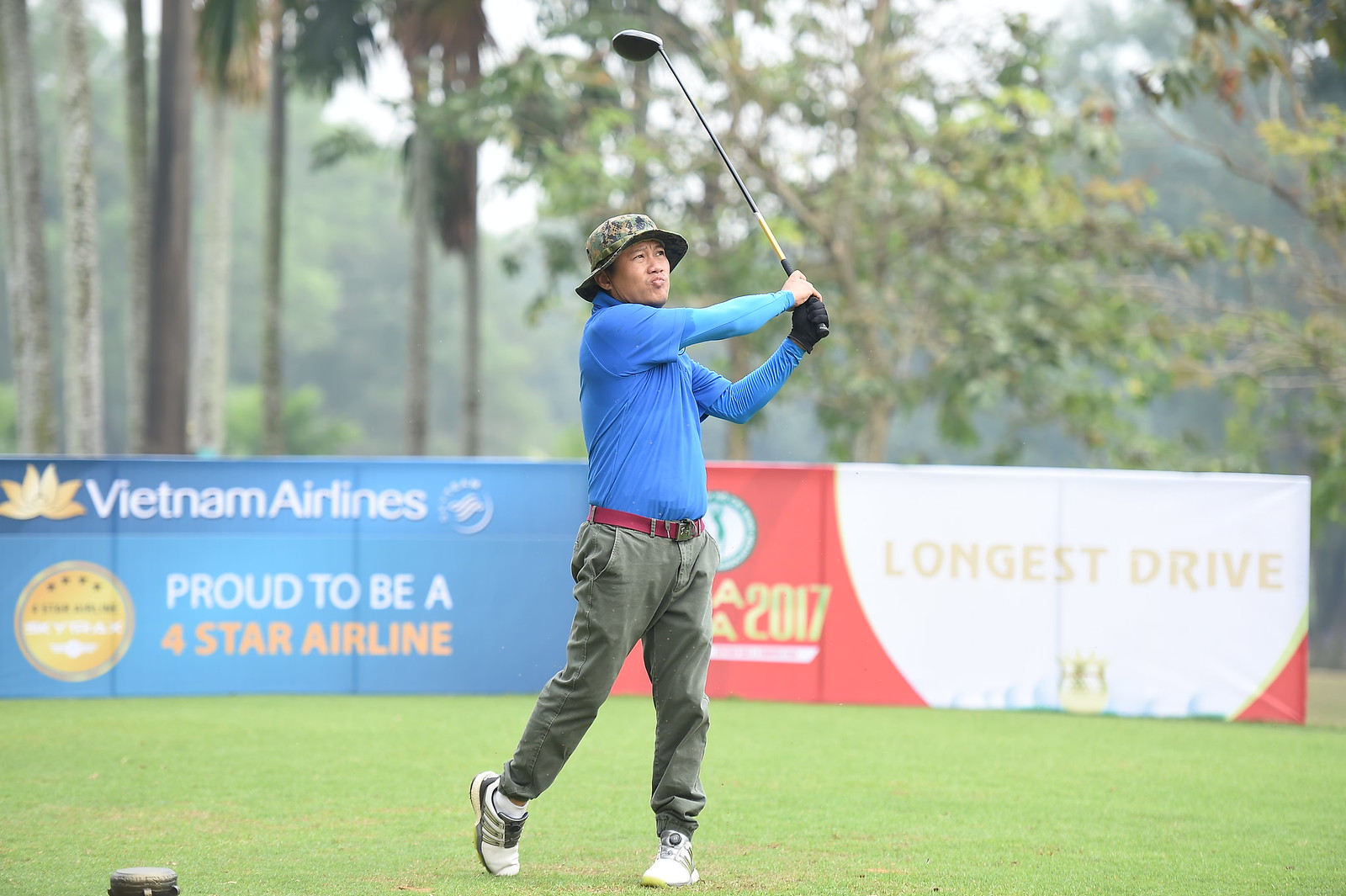The image depicts a man who just completed a golf swing, captured mid-pose on a lush green tee box. He is dressed in olive-colored pants, a long-sleeved blue golf shirt, and white golf shoes, accessorized with a red belt and a camouflage bucket hat. The golf club, a driver, is held high over his right shoulder. The background features a slightly overcast sky, with dense trees blurred in the distance. Several advertisement banners are visible; to the left, a banner reads "Vietnam Airlines, Proud to be a Four-Star Airline," colored in blue, white, and yellow, while to the right, another sign states "2017 Longest Drive" in red and white.